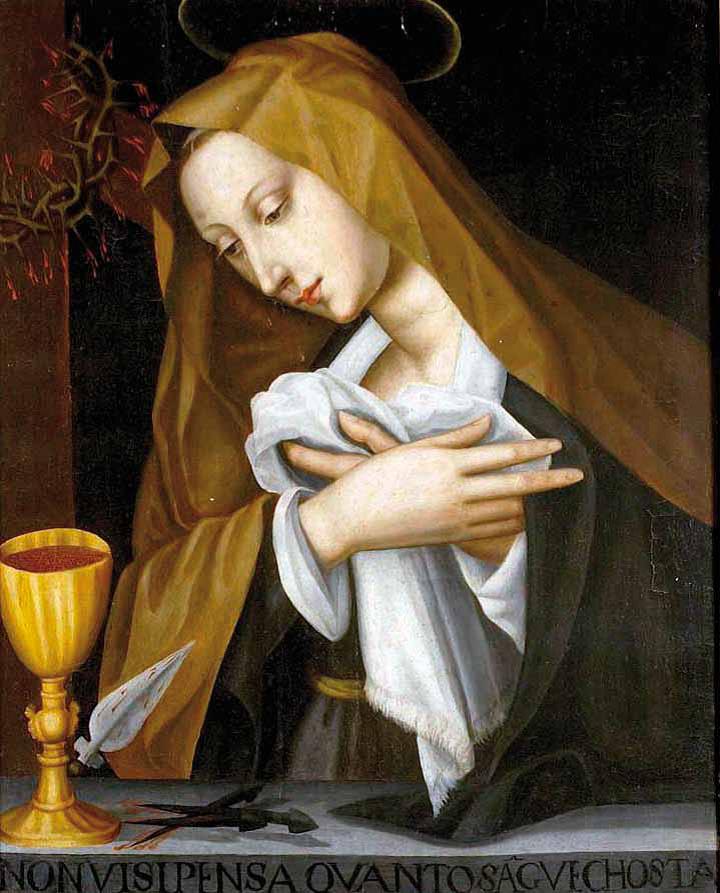The image depicts a religious painting by Plautilla Nelli, titled "Pained Madonna," characterized by a Mannerist style common in the late Renaissance. The portrait-oriented oil painting showcases a solemn woman who embodies saintly or biblical qualities. This figure, identified as a Madonna, is adorned with a halo and a crown of thorns, evoking strong religious connotations. She has light, porcelain-like skin and wears a golden-brown hood cascading down her shoulders alongside a dark green robe layered over a white undergown. A golden belt cinches her waist, complementing the neutral tones of her attire.

Seated at a table, she gazes downward at a gold chalice filled with a red liquid, symbolically reminiscent of blood or wine. Her arms are crossed over her chest, holding a white linen cloth. Accompanying her on the table are a prominent silver spearhead and several smaller black nails, further emphasizing the theme of suffering and sacrifice. The background is a stark black, accentuating the figure and the somber mood of the scene. At the bottom of the painting, an inscription in Latin reads "NON VICI PENSA O VANTO SAG VECOSTA," contributing to the artwork's profound spiritual and contemplative essence. The overall composition is richly detailed with hues of gold, red, maroon, and olive, enhancing the narrative of the depicted sanctity and sorrow.